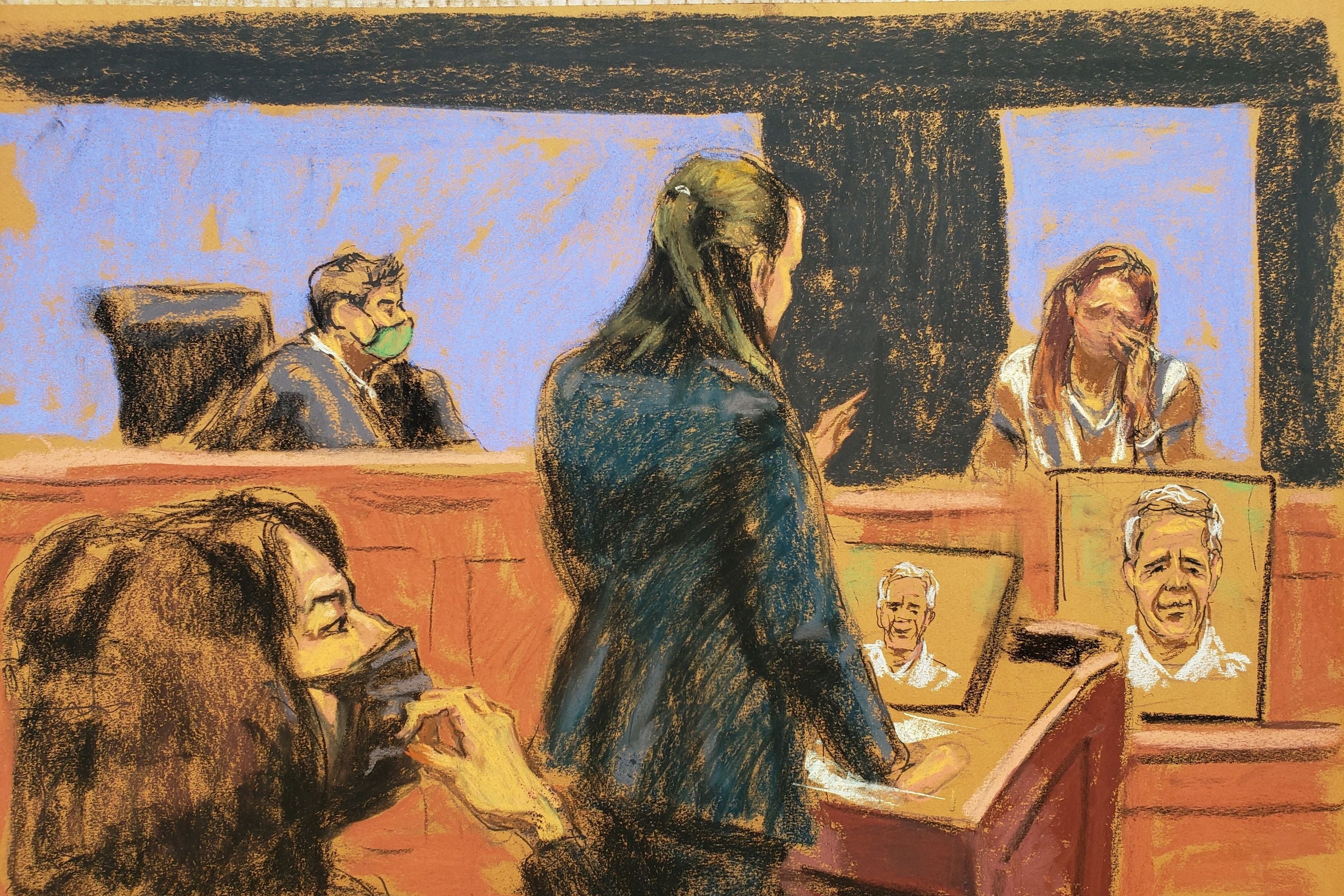The image is an artist's rendering of a courtroom scene, vividly illustrating the emotional intensity of the proceedings. In the foreground, on the left, a Caucasian woman with brownish hair and a face mask is depicted, her hand raised to the mask in a gesture of concern. She appears to be seated with her back almost to the audience, partially facing a woman in a dark navy blue blazer. This second woman, likely either the prosecutor or defense attorney, has long hair pulled back in a clip, with some strands pulled forward over her shoulders. She stands at a lectern, displaying a photograph of an older man with gray hair.

Center stage is the witness stand, where a woman appears to be crying, her head bowed and one hand covering her face, her longish hair draping around her. A large photo of the same older man from the lectern is prominently displayed in front of her. The judge, seated behind a reddish wood-colored bench, is angled toward the witness. He is wearing a green COVID-style face mask and has dark hair. Behind him, the background features a black wall interspersed with blue elements resembling windows.

Another woman, possibly the defendant, is seated and also wearing a COVID-style face mask. She has dark hair and appears very concerned, with her hand up to her mouth. The overall scene captures the somber and tense atmosphere of the courtroom, emphasizing the gravity of the moment being depicted.